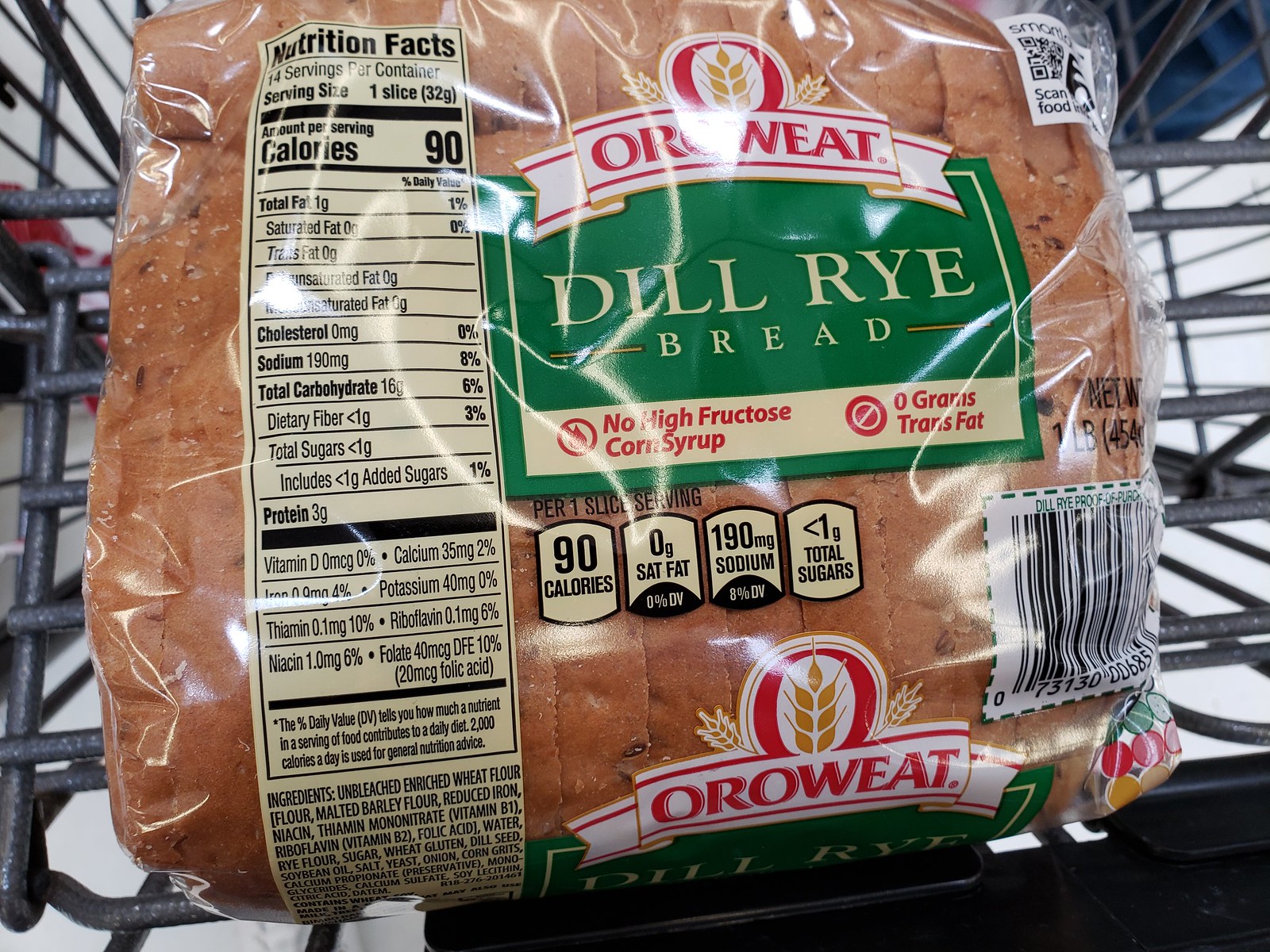In this detailed image taken inside a grocery store, we are looking down into a grocery cart, specifically the upper section designed for smaller items. The focus of the photograph is a close-up of a loaf of bread placed in this top compartment. The bread is branded as "Oroweat Dill Rye Bread," and the clear packaging prominently displays a variety of nutritional information. The labels, adorned in green, white, and red, indicate that the bread contains no high fructose corn syrup, zero grams of trans fat, 90 calories per slice, zero saturated fat, 190 milligrams of sodium, and less than a gram of sugar. On the right side of the packaging, a barcode is visible, while the left side presents a detailed tabulation of the nutritional facts. The metal grid of the grocery cart is also partially visible, contrasting with the bread's clear packaging.